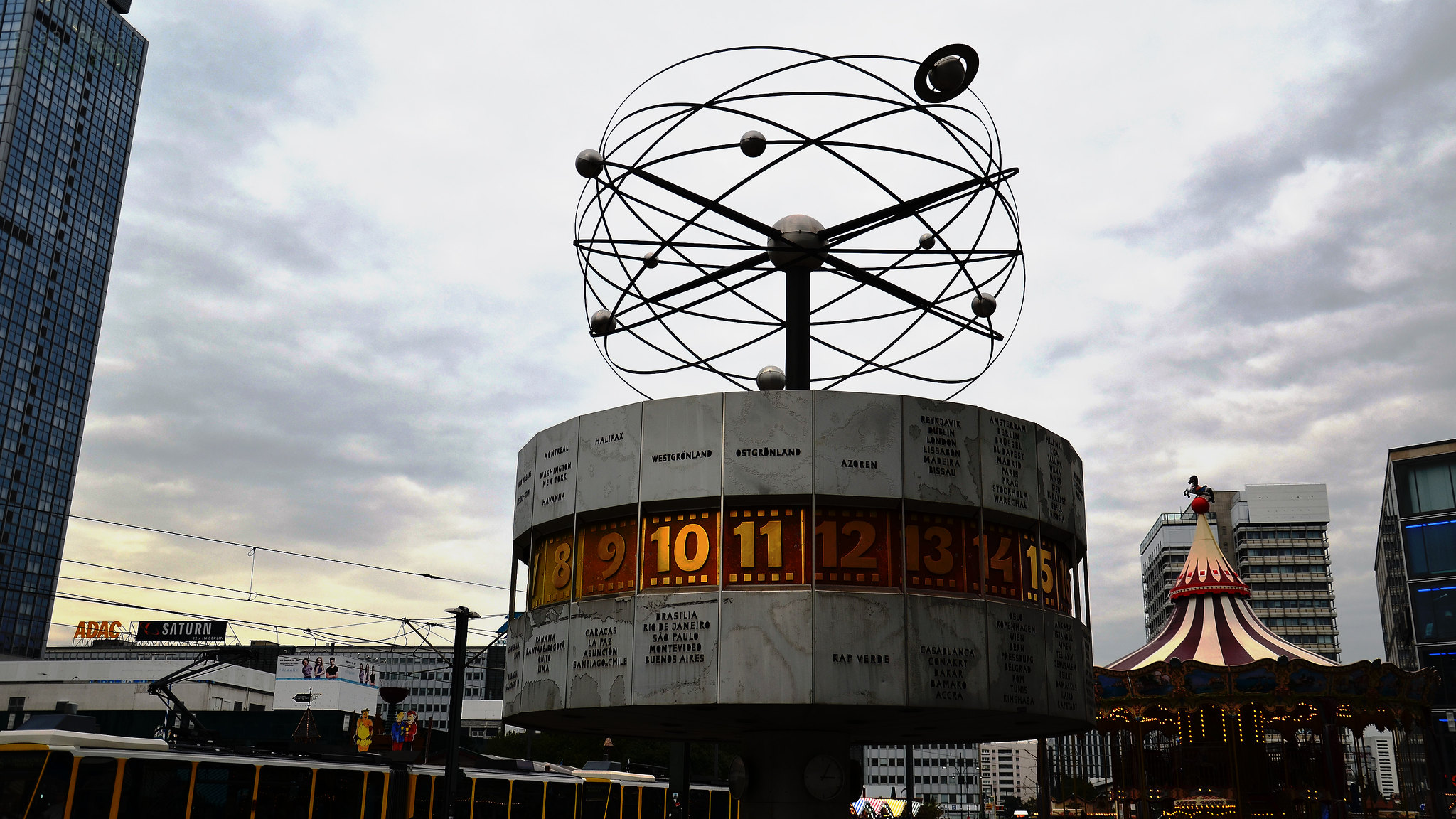The image depicts a prominent circular monument situated in a bustling urban area, possibly in Europe, known for its overcast, cloudy skies. This impressive structure, resembling a giant film roll or cylinder, features a series of gold numbers running sequentially from 8 to 15. Adorning its top is a striking metal sculpture, meticulously crafted to resemble a giant atom with interlocking silver rings and spherical nodes. Surrounding this central monument are various urban elements. To the left stands a blue glass skyscraper, approximately 25 stories tall, while additional buildings, including a 10-story and a 5-story structure, are visible in the background. On the right, a red-and-white striped carousel with a horse at its apex adds a whimsical touch. Other notable details include signs with "ADAC" and "Saturn" along with distant cable cars, indicating a vibrant, possibly fair-like environment. The overall atmosphere is one of a lively cityscape under a grey, cloud-laden sky.